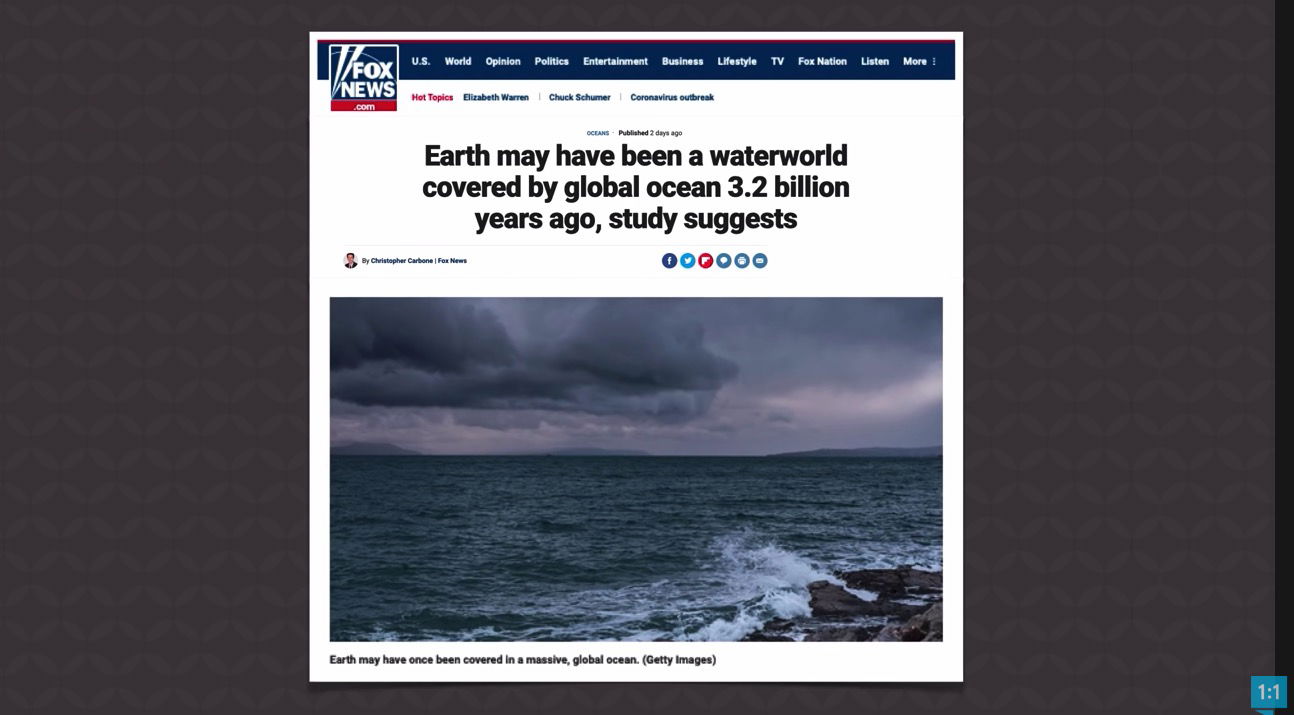The image features a detailed webpage screenshot with the following elements:

1. **Background Pattern**: Dominantly dark brown with a zigzag pattern interspersed with lighter brown.
2. **Main Screen**: A centered white section displaying Fox News content.
3. **Logos and Website Address**: The top left corner has the Fox News logo, and beneath it, the URL "foxnews.com".
4. **Navigation Bar**: A blue strip along the top lists navigation links including U.S., World, Opinion, Politics, Entertainment, Business, Lifestyle, TV, Fox Nation, Listen, and War.
5. **Hot Topics Section**: Below the navigation bar, a white background area lists "Hot Topics" in red, with topics like Elizabeth Warren, Chuck Schumer, and Coronavirus Outbreak in blue or black text.
6. **Recent Article**: An article published two days ago mentions, "Oceans: Earth may have been a water world covered by global oceans 3.2 billion years ago, study suggests."
7. **Article Image**: There’s a photograph depicting a vast ocean under dark, cloudy skies with a hint of pinkish light breaking through, creating a dramatic atmosphere over the dark blue-green water with visible white splashes.
8. **Additional Annotations**: The article appears to be credited to Christopher Carbon and includes notes about "Free News" and mentions that "Earth may have once been covered by a massive global ocean," according to Getty Images.

Overall, the image highlights a Fox News webpage with prominent navigation, current hot topics, and an article discussing ancient global oceans, accompanied by a visually striking photograph.